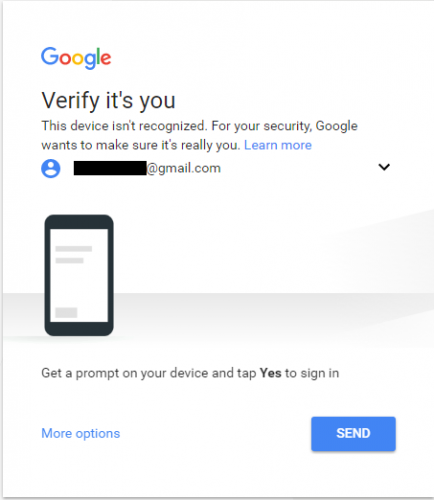The image features a clean white background with a gray border framing the top left and bottom edges. At the top center of the image, the Google logo is prominently displayed, comprised of two blue "G"s, a red "o", a yellow "o", a blue "g", a green "l", and a red "e". Directly beneath the logo, in large, black, bold letters, are the words "Verify It's You."

Below this header, the text reads, "This device isn't recognized. For your security, Google wants to make sure it's really you." Accompanying this message is a blue hyperlink labeled "Learn more." 

Beneath the explanatory text is a blue generic default profile picture. A black box obscures a portion of the text, leaving only the "@gmail.com" suffix visible to its right.

To the right of this obstructed text, there is an icon depicting a tablet. The tablet is outlined in black with a white screen, showing two gray lines at the top and one at the bottom. Below the tablet icon, the instructions state, "Get a prompt on your device and tap Yes to sign in."

At the bottom-left of the image, another blue hyperlink reads "More options." Adjacent to the hyperlink, a rectangular-shaped blue button is labeled "Send."